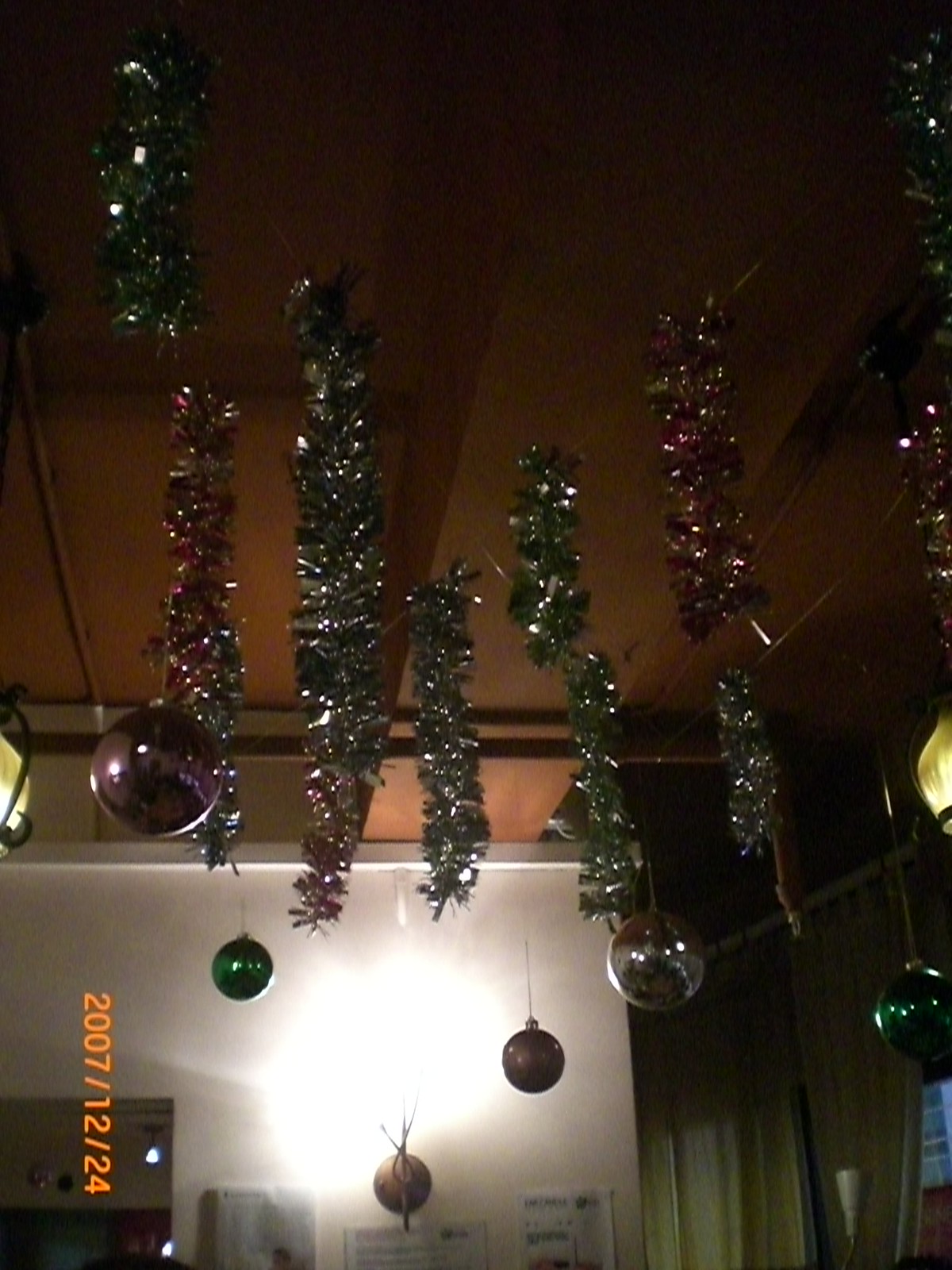This color photograph, taken indoors under low light conditions, captures the ceiling of a large function hall lavishly adorned with Christmas decorations. The camera is angled upward, pointing towards the tall, smooth brown ceiling, which features a centrally positioned white light. Suspended from the ceiling, though the wires are not visible, are various strands of shiny tinsel typically used to decorate Christmas trees. The tinsel exhibits festive red and green hues, intricately mixed with silver segments. Hanging slightly lower than the tinsel are reflective glass baubles, also in thematic colors of red, maroon, green, and occasionally purplish tones, all glimmering in the low light. 

In the lower left corner of the image, an orange date stamp—"2007/12/24"—is oriented vertically, indicative of the photo being taken on Christmas Eve. The background reveals a green curtain on tracks in the back right corner, which likely serves as a room divider or to block windows, adding to the festive yet functional ambiance. This scene appears to be set in a sizable venue, as suggested by the tall ceiling and the green fabric curtains concealing parts of the space, contributing to its cozy and decorated aesthetic.